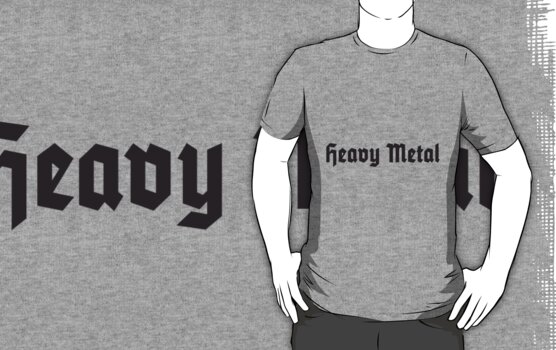This image is a digitally created, black-and-white line art illustration with a gray background. Positioned off-center to the right, the illustration features a man facing the viewer, depicted from below his chin down to his hips. He is wearing a gray t-shirt with dark gray pants, and his hands are in his jeans pockets. The t-shirt has the words "Heavy Metal" emblazoned across the chest in a gothic black script. The man's skin, which includes his arms, neck, and face, is illustrated in white. To the left of the man, partially cut off, is the word "Heavy" in large black letters. The background behind the man features close-up details of the same "Heavy Metal" logo on his shirt, incorporating torn fabric and metal elements. The overall composition suggests this might be an advertisement for either a t-shirt or a musical group, emphasized by the monochromatic color scheme consisting of various shades of gray, black, and white.